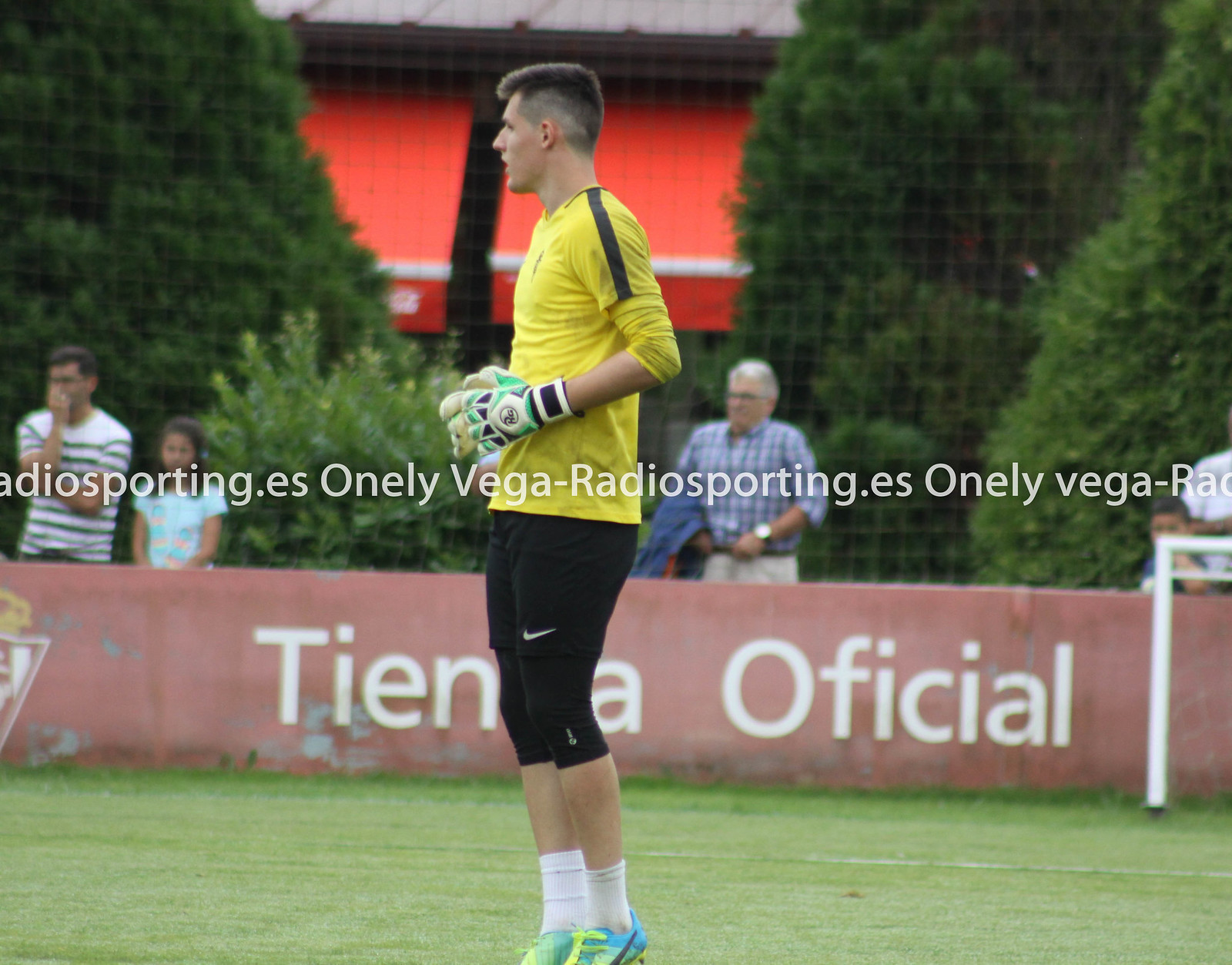The photograph captures a soccer player standing on a green grassy field, depicted in a horizontal rectangular format. The player, situated centrally, is seen from the side. He is dressed in a yellow t-shirt paired with knee-length black shorts and large green gloves, suggesting he is likely a goalkeeper. Surrounding him is the expansive green field. In the background, there is a brown fence adorned with large white text that reads "Tiana official." Behind the fence, a group of spectators is visible, including a man in a striped shirt with glasses and a hand on his face, a little girl in a floral dress, and an older man with white hair, a blue shirt, white pants, and a watch holding a jacket. Further back, the scene is framed by lush green trees and an orange pavilion. Additionally, there is a watermark across the middle of the image displaying the text "onlyvegaradiosporting.es."